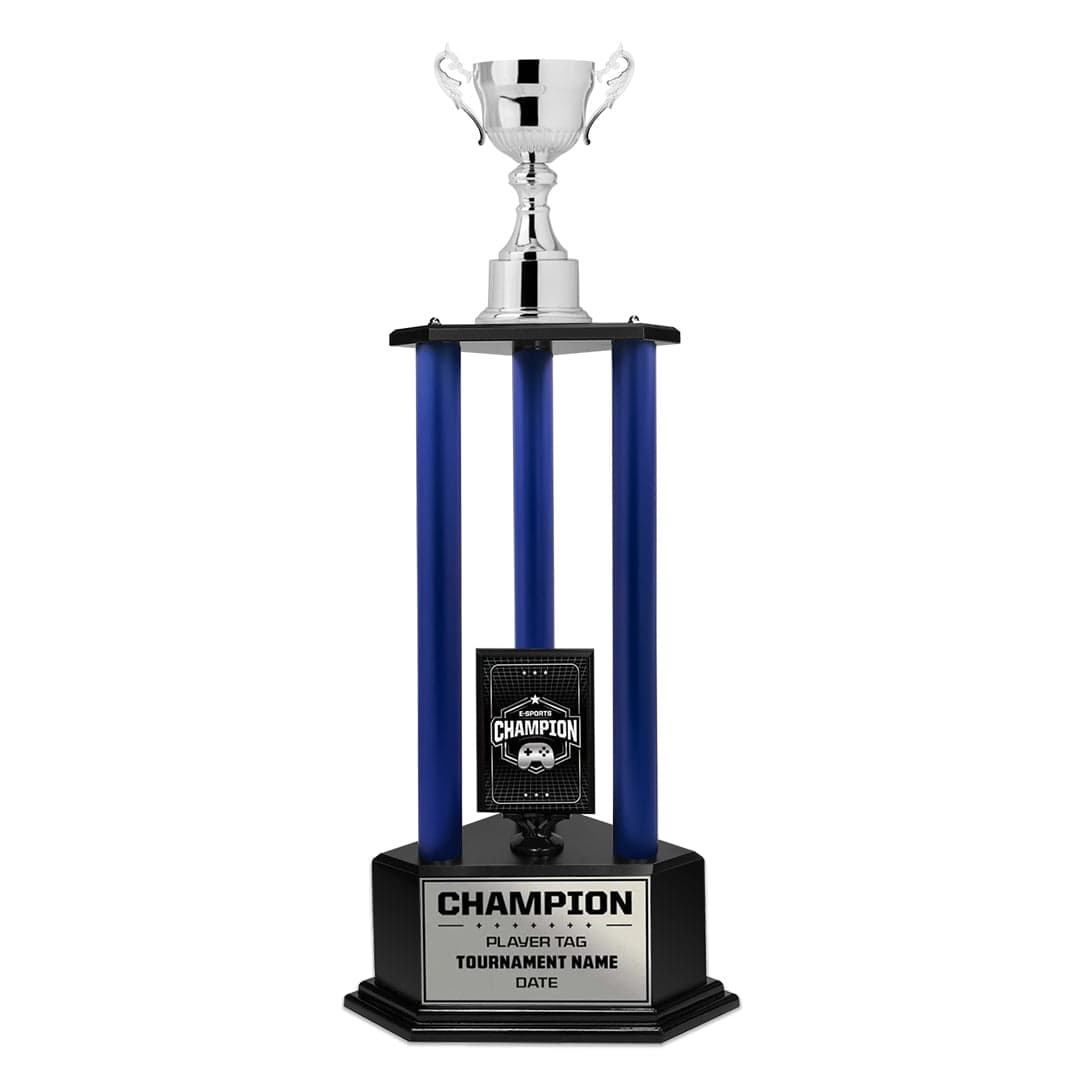This is a photographic image depicting a silver trophy with a white background, suggesting it's taken indoors. The trophy features a classic design with a polished silver cup, ornate curved handles on either side, and a sturdy structured base. The base itself is triangular, with three tall, shiny blue metal columns arranged in a triangular layout supporting a black platform. Centrally placed on the base is a silver plaque that reads "Champion," followed by fields for a player tag, tournament name, and date, with the plaque bordered by a black frame and a distinctive lip at the bottom.

Additionally, between the three blue columns, there is a black card marked "Sports Champion" in white letters. The card displays a logo consisting of a star and a video game controller, indicating the trophy is likely intended for an eSports tournament. The entire presentation suggests it is a promotional image of a customizable team trophy, captured in a portrait orientation.